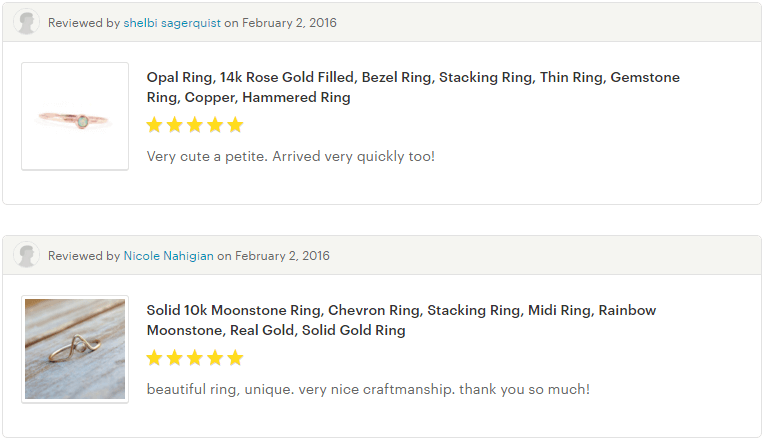At the top of the image, there is a light gray strip bordered by a darker gray. On the left side of this header, a circular icon with a gray border features the silhouette of a man looking sideways to the right. Adjacent to this icon, the text "Reviewed by" is presented in black, followed by "Shelby Sagerquist" in blue. Further to the right, in black text, the date is listed as "February 2, 2016."

Beneath this header is a white rectangular section. On the left side of this area, an image displays a copper ring with a circular diamond set in the middle. To the right of the image, detailed product information reads: "Opal Ring, 14K Rose Gold Filled, Bezel Ring, Stacking Ring, Thin Ring, Gemstone Ring, Copper, Hammered Ring." Below this description, five yellow stars indicate a rating, and beneath these stars, a small dark gray review says, "Very cute. Petite. Arrived very quickly!!"

At the bottom of the image, there is another white rectangular section. On the left side of this bottom section, an image showcases a moonstone ring. To the right, the heading reads: "Solid 10K Moonstone Ring, Chevron Ring, Stacking Ring, Midi Ring, Rainbow Moonstone, Real Gold, Solid Gold Ring." Below this caption, five yellow stars are displayed once again, indicating another rating.